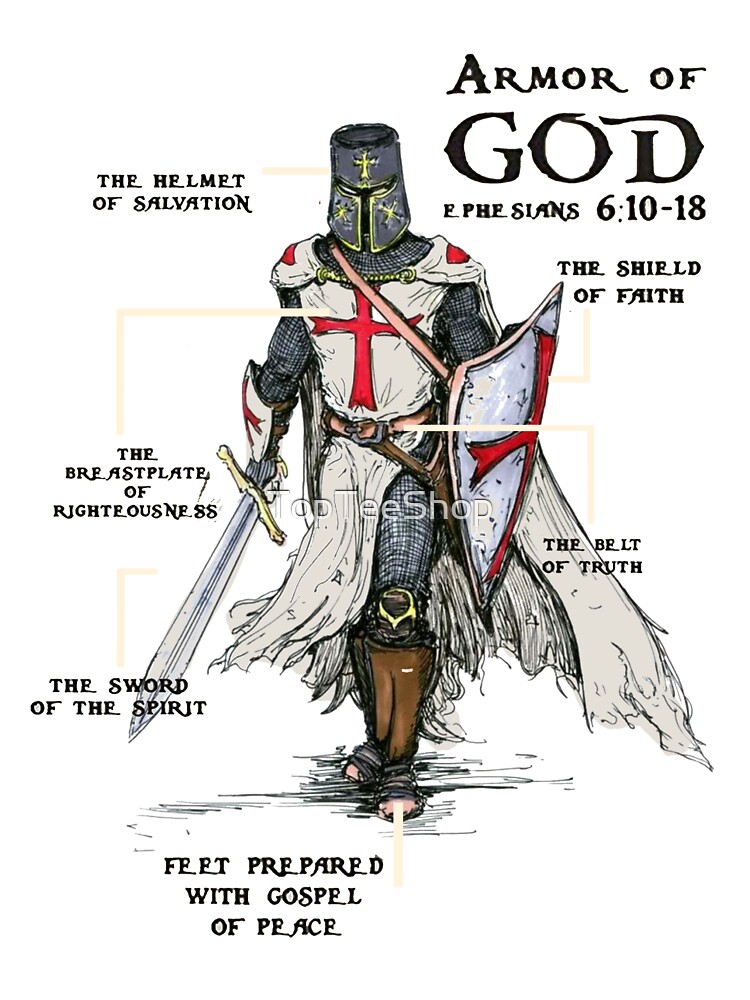The illustration is an informative diagram titled "Armor of God" with a reference to Ephesians 6:10-18 in the top right corner. The drawing features a medieval knight adorned in religiously symbolic armor. The knight wears a gold and blue helmet with crosses, labeled as the "Helmet of Salvation." The knight's outfit is predominantly white with red crosses, featuring a breastplate labeled the "Breastplate of Righteousness." Brown boots and knee guards complete the attire, with the feet labeled "Feet prepared with the Gospel of Peace." In the knight's right hand, there is a large sword labeled the "Sword of the Spirit," and in the left hand, a white shield with a red cross labeled the "Shield of Faith." The diagram also points out a belt, labeled the "Belt of Truth." The detailed labels and arrows provide a thorough explanation of the different components of the armor, integrating both visual and textual descriptions to convey the metaphorical 'Armor of God'.